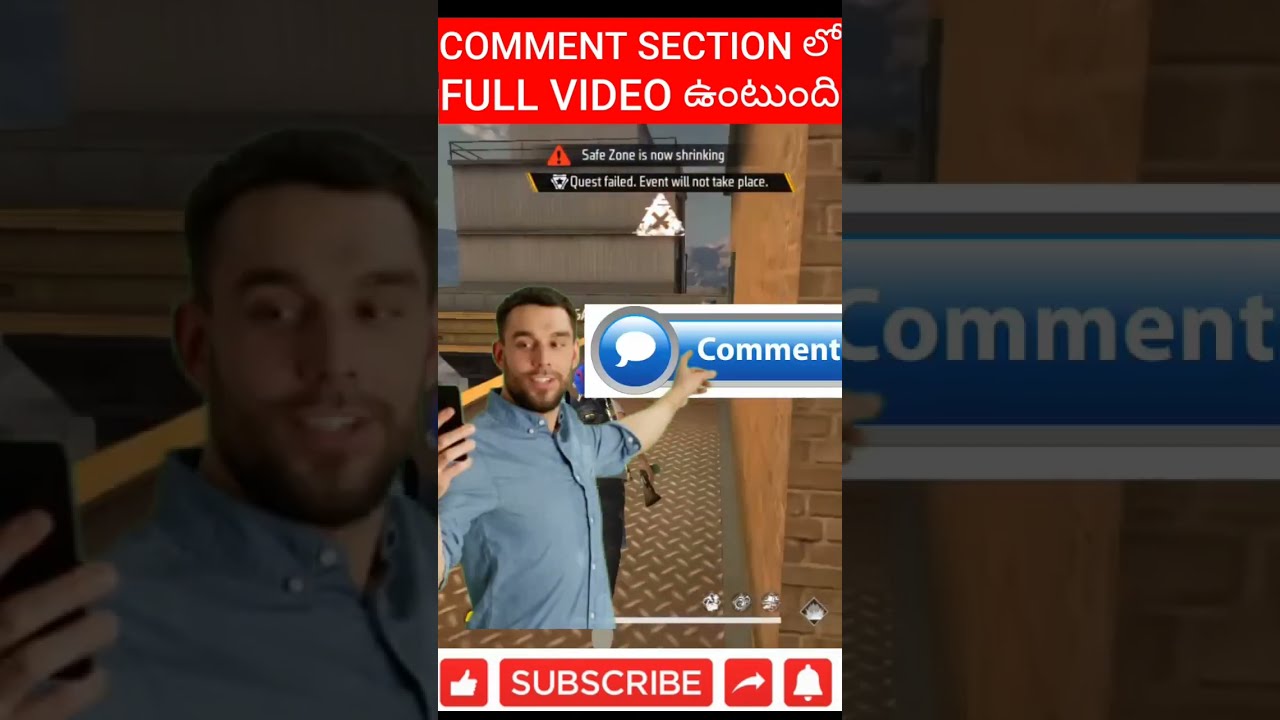The image features a young man in a blue collared short-sleeved shirt pointing to the comment section on the image. At the top, there is a bold red band with the text "COMMENT SECTION FULL VIDEO" in white. Below this, in white text, it states "SAFE ZONE IS NOW SHRINKING, QUEST FAILED, EVENT WILL NOT TAKE PLACE," suggesting a video game backdrop. The background is a computer-generated scene with a brick wall, a steel floor, and metal rails. At the bottom of the screen, there is a white bar with various icons, including a thumbs-up in a red box, a 'subscribe' button, a save icon, and a notification bell. The man appears to be holding a phone and pointing towards a text box with the word "COMMENT" and a comment bubble beside it, indicating interaction with the comment section in what seems to be a live stream or a video screenshot.